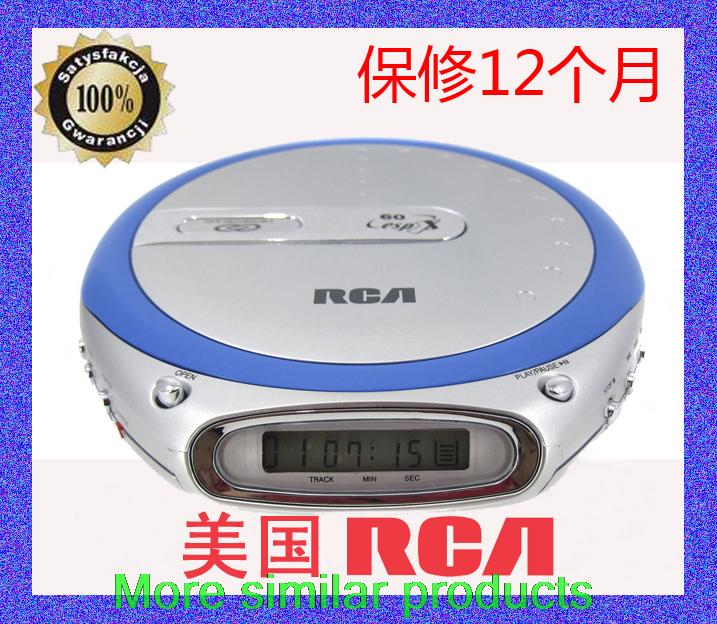This image depicts a detailed advertisement for a silver and blue RCA CD player, reminiscent of the CD alarm clocks popular in the 1990s and early 2000s. The product is prominently featured in the center of the ad, encased in a blue confetti-style frame against a white background. The CD player includes a digital display that indicates track, minutes, and record functions, suggesting it is equipped for music playback and possibly radio. Noteworthy elements include two buttons on top labeled "open" and "play/pause." 

The branding, RCA, is prominently displayed both on the CD player and in large red letters within the ad, which is primarily written in an Asian language, possibly Korean or Japanese. The top left corner features a gold seal with a black circular band containing Asian characters and "100%" in the center, indicating a satisfaction guarantee. Meanwhile, the top right corner shows additional red Asian writing with the number "12" and an up arrow. The bottom center of the ad includes more Asian symbols in red, and in green lettering, it offers information about similar products, indicating the availability of other electronics.